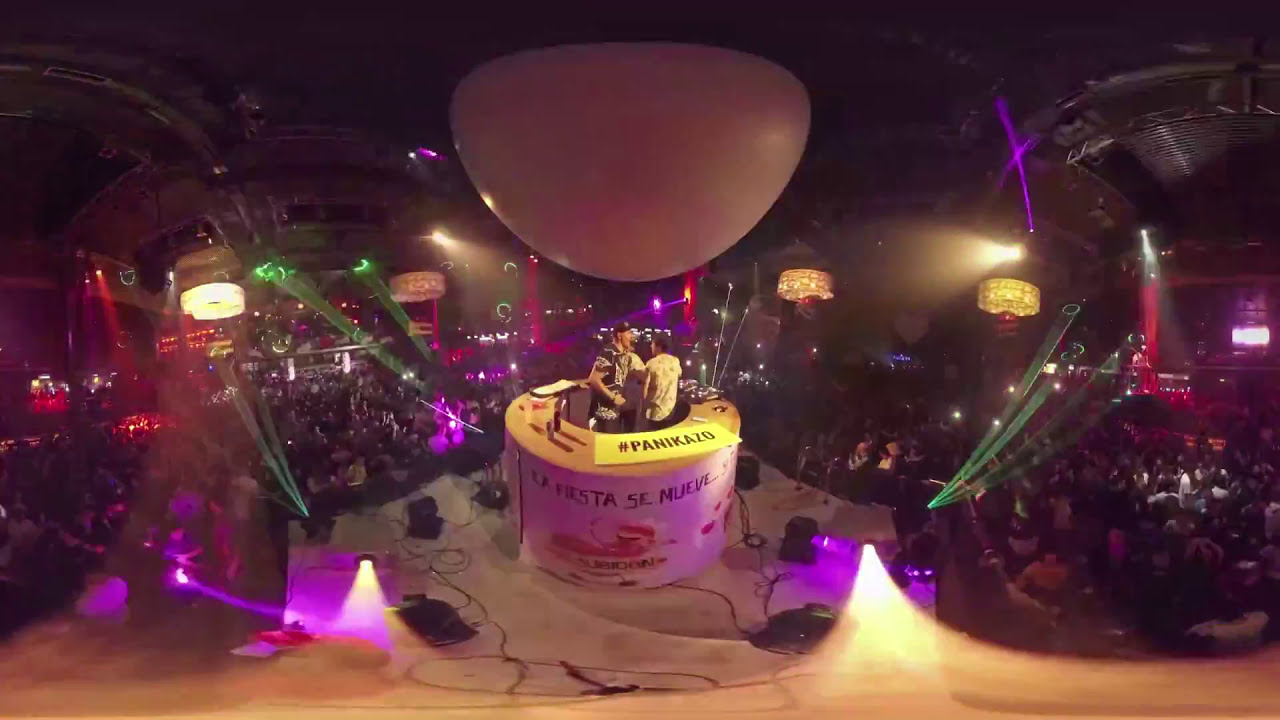The image depicts a rectangular, horizontally oriented stage inside what appears to be a nightclub, engulfed in an atmospheric, dark background. The focal point is a pair of men standing in a hollowed-out, tan cylinder on the stage. The cylinder, a few feet tall, has a sign on its exterior that reads "La Fiesta Se Nueve" in black, and features a yellow, rectangular label on top with "Panticazo" also in black. A unique dome-shaped cover, white in color and resembling an upside-down dome, appears to float above the booth, with no visible supports. The stage, adorned with small black lights, speakers, and electrical cords, is surrounded by multidirectional strobe lights emitting green, purple, red, and yellow hues. In the background, a sizable, engaged crowd gazes up at the stage, with silhouettes of people visible. This lively scene suggests the men could be DJs performing at a bustling concert or nightclub, underscored by the presence of the strobe lights and audience below.